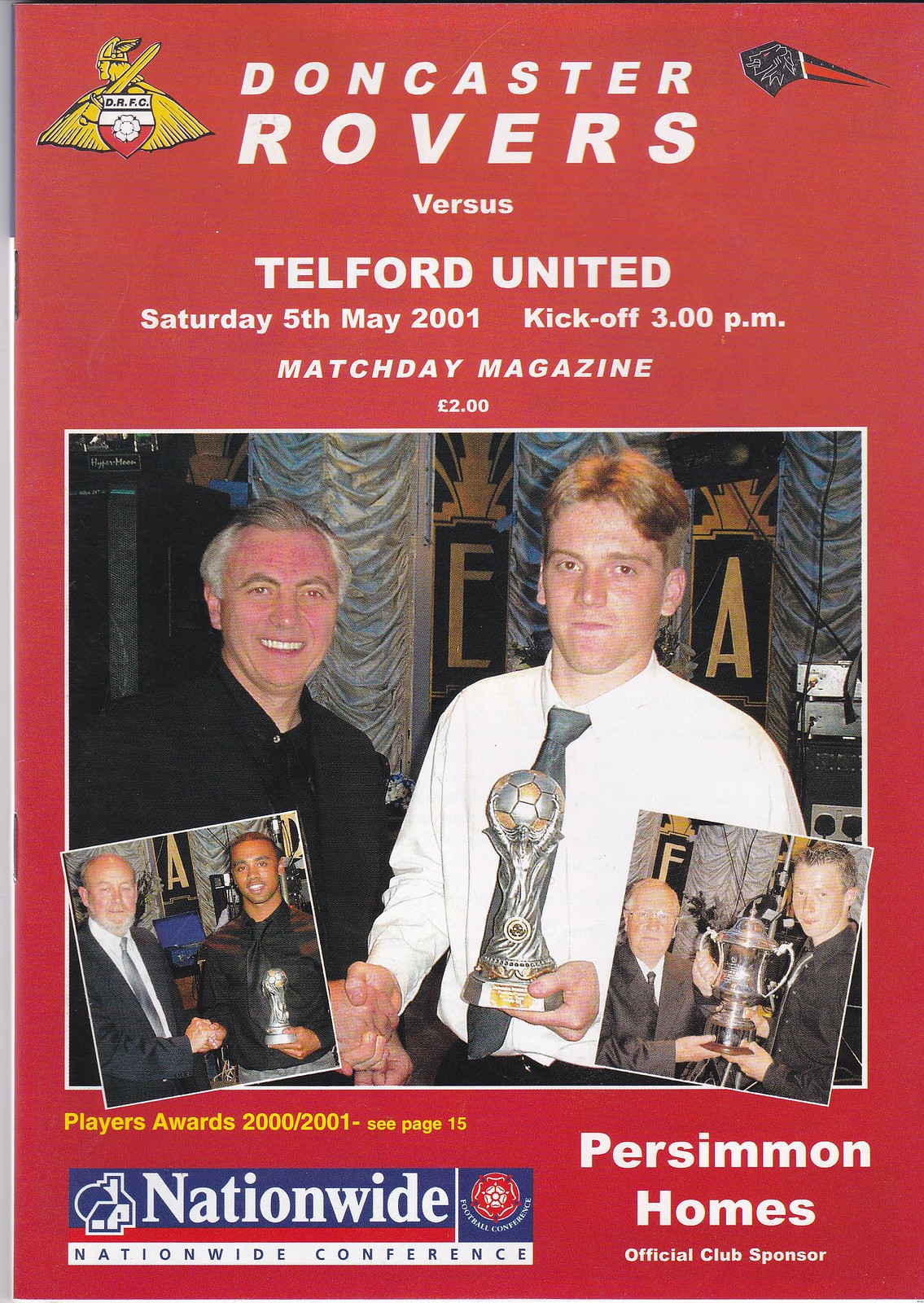This detailed caption shows a program guide for an English Football League match between Doncaster Rovers and Telford United, which took place on Saturday, May 5, 2001, with a kickoff at 3 p.m. This Matchday Magazine, priced at two pounds, features a vibrant red cover with a yellow symbol on the upper left side and a black symbol on the right. The magazine prominently advertises the Player Awards for the 2000-2001 season on page 15 and mentions the Nationwide Conference with Persimmon Homes as the official club sponsor.

On the cover, two main figures are depicted: an older man in a black shirt standing on the left, and a younger man in a white dress shirt with a black tie on the right, who is holding a trophy. Below these main images, there are two smaller photographs. One shows a young man in a black shirt receiving an award, and the other is of another individual in a suit. These images collectively highlight the various recipients of awards, celebrating their achievements. The background of the cover is a bold burgundy, accentuating the prominence of the figures and text. Overall, the magazine captures the significance of the upcoming matchday and the celebration of player achievements.